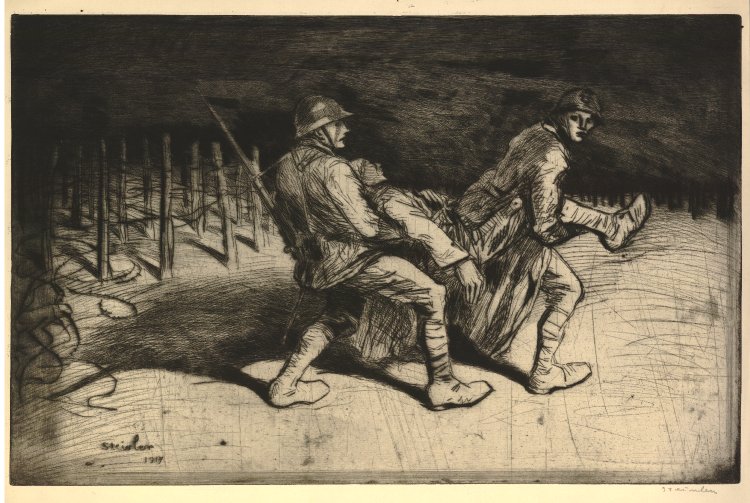The artwork portrays a dramatic World War I scene, illustrated predominantly in pen and ink with hues of gray and beige. Central to the image are two soldiers, each donning an army helmet, struggling to carry a wounded comrade. The soldier at the back, identifiable by the rifle strapped to his back, lifts the injured man by his shoulders, his face marked by terror. In contrast, the soldier at the front, clad in a trench coat, carries the man's legs while anxiously glancing back towards his partner. Their legs are bent under the weight, indicating the strain of their task. The composition is bisected by a strong light source on the right, casting deep shadows to the left. Background details, including barbed wire fencing on posts, reinforce the wartime context while a dark, textured sky looms above a lighter ground, adding to the sense of urgency and foreboding.